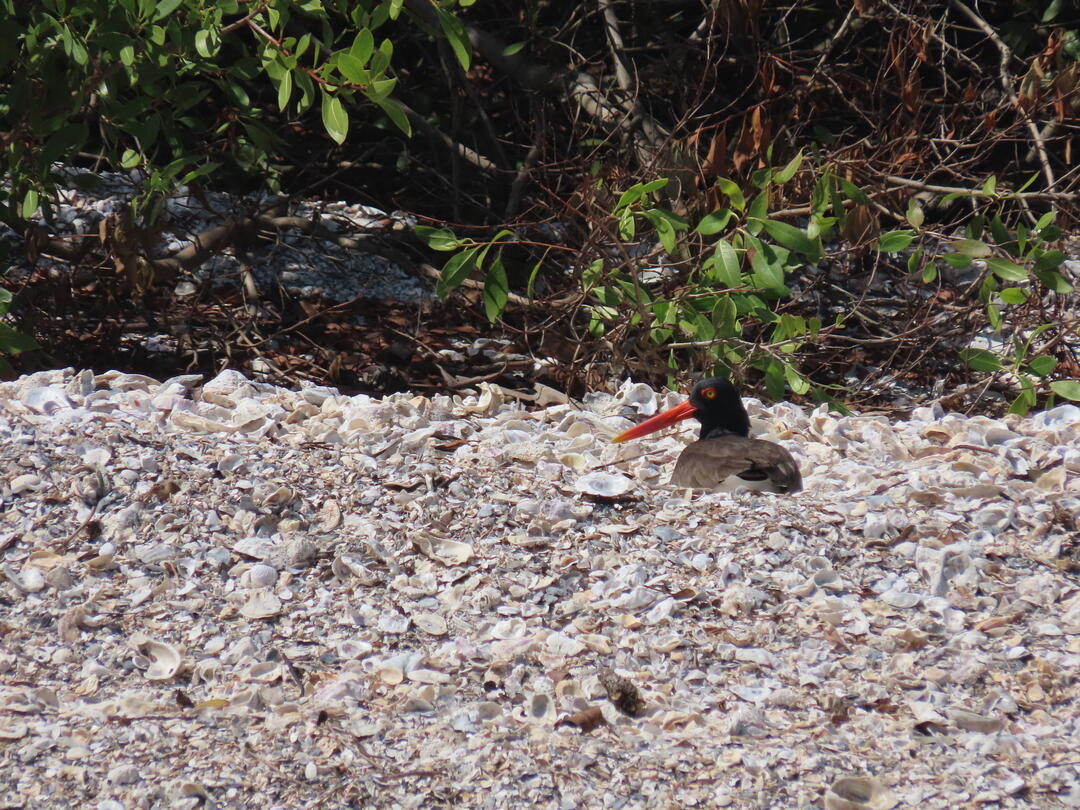The image appears to be an edited or AI-generated photograph taken at what could be a beach setting. The ground in the foreground is strewn with debris resembling broken shells, shells, or garbage, displaying a mix of white, light tan, and gray tones. Situated among this debris is a bird with a long orange beak that turns yellow at the tip, and an orange eyebrow stripe. The bird's head is black, the body transitions to gray, and it also features a visible white underbody. The eye is ringed with red skin, adding to its striking appearance. Only the upper half of the bird’s body is visible, leading to speculation that the lower half might be buried in the shells or skillfully edited out. The background consists of primarily small branches and green foliage, with some areas showing dead or missing leaves. The daylight lends a natural brightness to the scene, highlighting the bird facing left and suggesting a somewhat surreal or artistic composition.